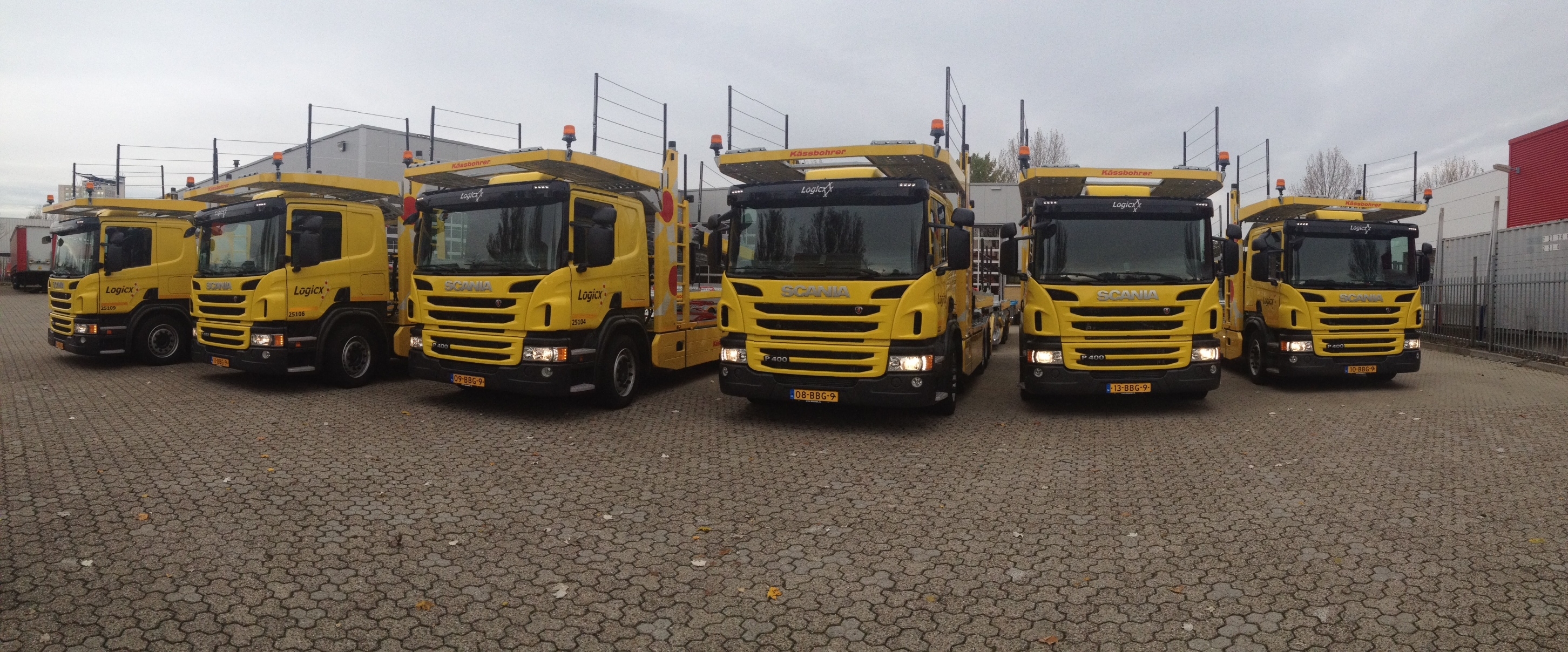This outdoor photograph captures a fleet of six identical yellow flatbed European work trucks arranged in a fan-like formation. Four of the trucks are visible from the front, and two from a front-side angle. Distinctive features of the trucks include black windshields, black frames, and a flat yellow piece that covers the top of the cube-shaped cabs, which also have a platform with wire railings and two orange lights. The trucks are parked on a light brown-gray surface made of interlocking three-sided tiles, resembling puzzle pieces. In the background, the scene includes a partial view of a concrete building on the top left and a combination of metal rectangles with horizontal wires on the right side. The sky is cloudy, casting a gray hue over the image.